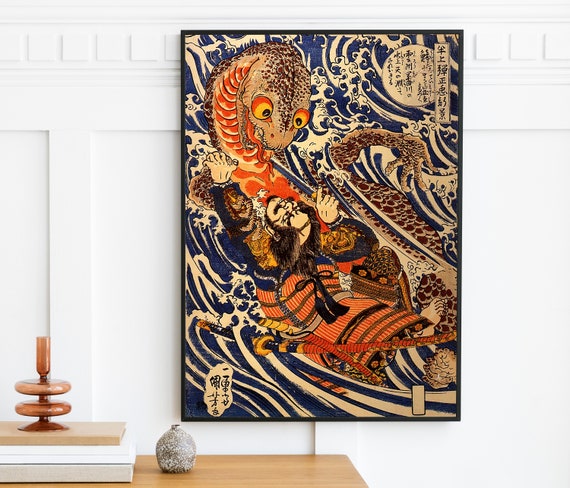A staged photograph showcases a white wall adorned with detailed molding, giving the impression of larger and smaller rectangles set within the wall. The focal point is a Japanese-style painting hanging prominently on the wall. The painting, rich in East Asian artistry, likely Japanese, illustrates an intense battle between a man and a sea monster. The background bursts with swirling blues and ivory stripes, accentuating the drama. The sea monster, with its red, orange, and yellow eyes against dark, scaly skin, is depicted lying on its back, exposing its orange underbelly and claws emerging from the water. The man, characterized by his bald top and hair on the sides, complete with a bushy mustache and poofy eyebrows, grapples with the monster’s fin while looking fiercely into its eyes, teeth gritted. He's clad in armor, donning a blue top and a red and yellow striped sash, with two sheathed swords at his side, adding to his warrior persona. The scene is framed by Japanese text situated in the top right and bottom left corners of the painting.

A light to medium brown wooden table partially visible in the bottom left corner of the photo supports a small collection. On it sits a trio of books – grey, white, and beige in descending order – topped by a clear, brown glass vase. This vase features a unique design with a circular base leading up to a champagne flute-like slender glass top. Beside it stands a smaller, gray stone vase. The combined elements create a detailed, immersive setting, embedding the artwork deeply into its environment.